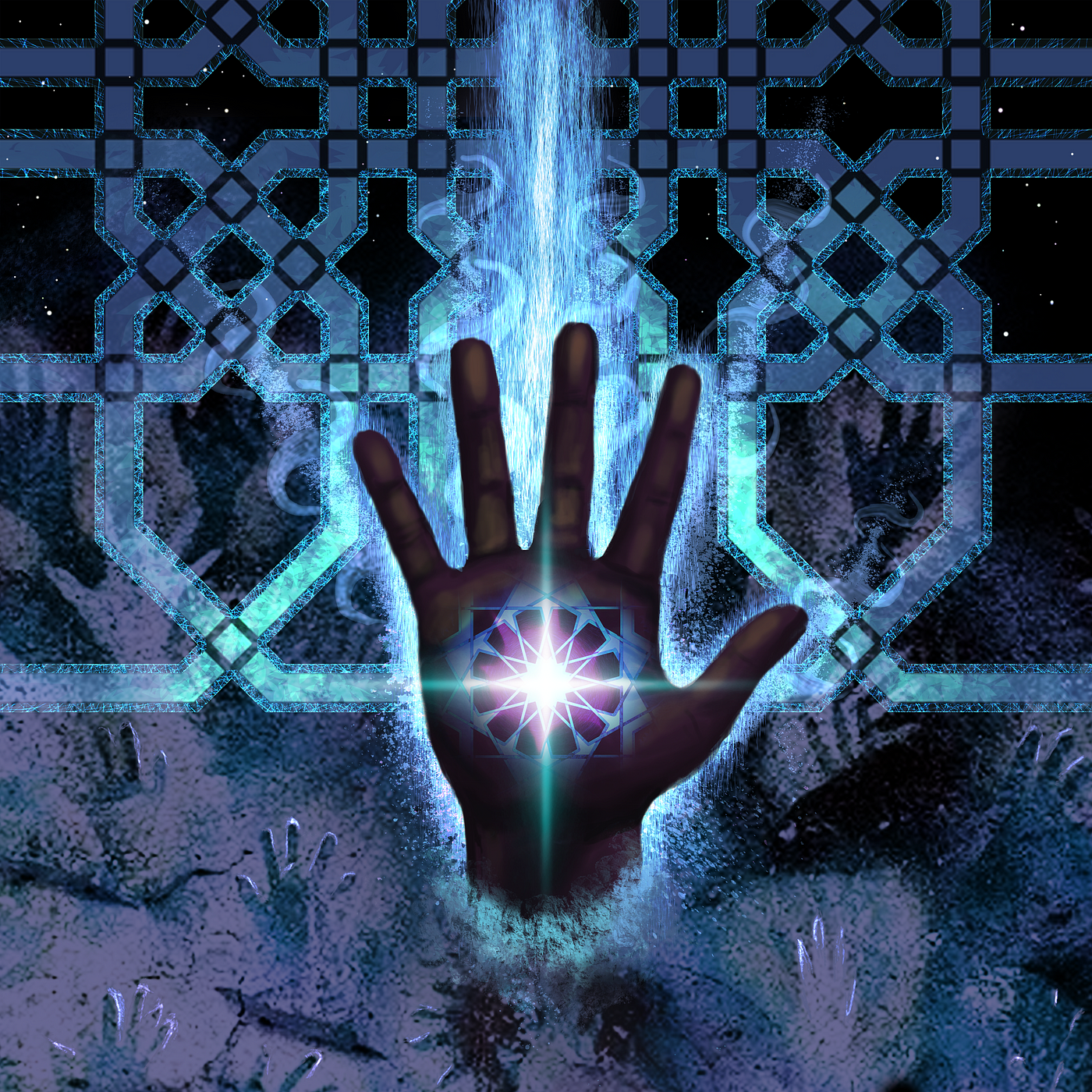This image is a captivating and mysterious artwork centered around an outstretched dark-colored hand. The hand, facing towards the viewer with its palm open, features an ornate, star-like shape that emits a radiant white glow. This intricate design within the palm appears almost floral and is surrounded by beams of light extending outward. The background is a dark, textured blend of purples and blues, adding to the eerie, enigmatic atmosphere.

Behind the hand, a prominent, glowing vertical shape shoots upward, adorned with geometric, maze-like patterns that contribute to the surreal and dreamlike ambiance. Surrounding this central hand are faded, ghostly silhouettes of other hands, reaching up as if emerging from an abyss, enhancing the image's haunting quality. The upper portion of the background mimics a night sky with tiny dots resembling stars, further enriching the scene with a celestial touch.